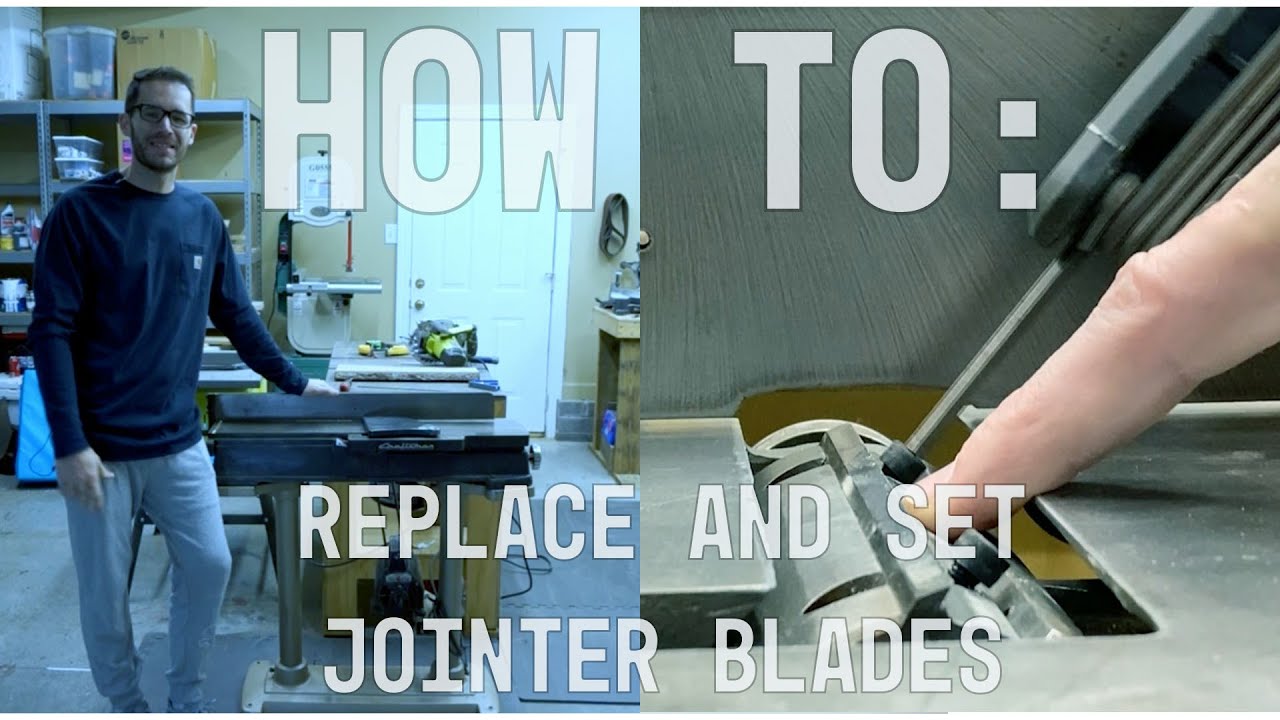In the detailed photo, a step-by-step guide on "How to Replace and Set Jointer Blades" is prominently highlighted, with the phrase spelled out in block letters. The central figure is a man dressed in a black long-sleeve shirt and blue pants, accessorized with glasses. He is positioned beside a piece of machinery located in the middle of the room. His left hand rests on the machinery, indicating the focus of the replacement process. 

The backdrop includes a gray rack filled with various boxes and tubs, suggesting a well-organized workspace. To the right of the image, a wooden table and a white door are visible, set against a concrete floor which adds an industrial feel to the scene.

On the right side of the photo, a close-up reveals the man holding a cylindrical component with a sharp blade, positioned carefully with one finger. Adjacent to this, an Allen key set is shown actively turning a screw, illustrating a part of the maintenance process involved in blade replacement. This detailed capture provides a comprehensive view of both the workspace environment and the technical steps for setting jointer blades.